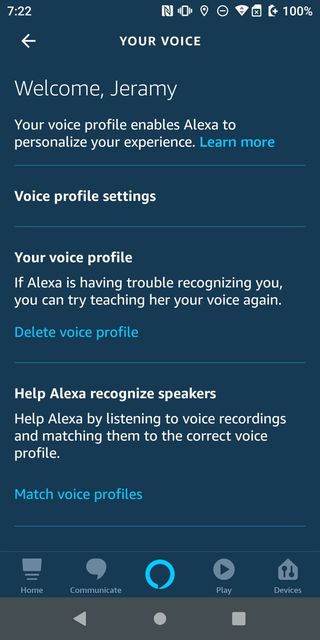This is a detailed and cleaned-up caption for the given screenshot:

---

The screenshot, captured from an Android phone, showcases the Alexa app interface with a dark blue background and predominantly white text. At the very top, the notification bar displays the time as "7:22" on the left, along with various status icons on the right, including battery, Wi-Fi, Do Not Disturb, location, and vibrate icons. 

Beneath the notification bar, the header of the app reads "Your Voice" centered at the top, with a back button located on the left. Directly below, a welcome message addresses the user: "Welcome, Jeremy. Your voice profile enables Alexa to personalize your experience." A clickable "Learn more" link in light blue appears next. 

The section labeled "Voice Profile Settings" follows, featuring an instructional note: "If Alexa is having trouble recognizing you, you can try teaching her your voice again." Another clickable link, "Delete Voice Profile," is provided in light blue. 

The lower part of the screen contains a segment titled "Help Alexa Recognize Speakers," explaining that users can assist Alexa by matching voice recordings to the appropriate voice profile. A clickable option, "Match Voice Profiles," is available.

At the very bottom, the app's navigation bar displays five buttons: "Home," "Communicate," an Alexa activation button represented by a circular icon in the center, "Play," and "Devices."

---